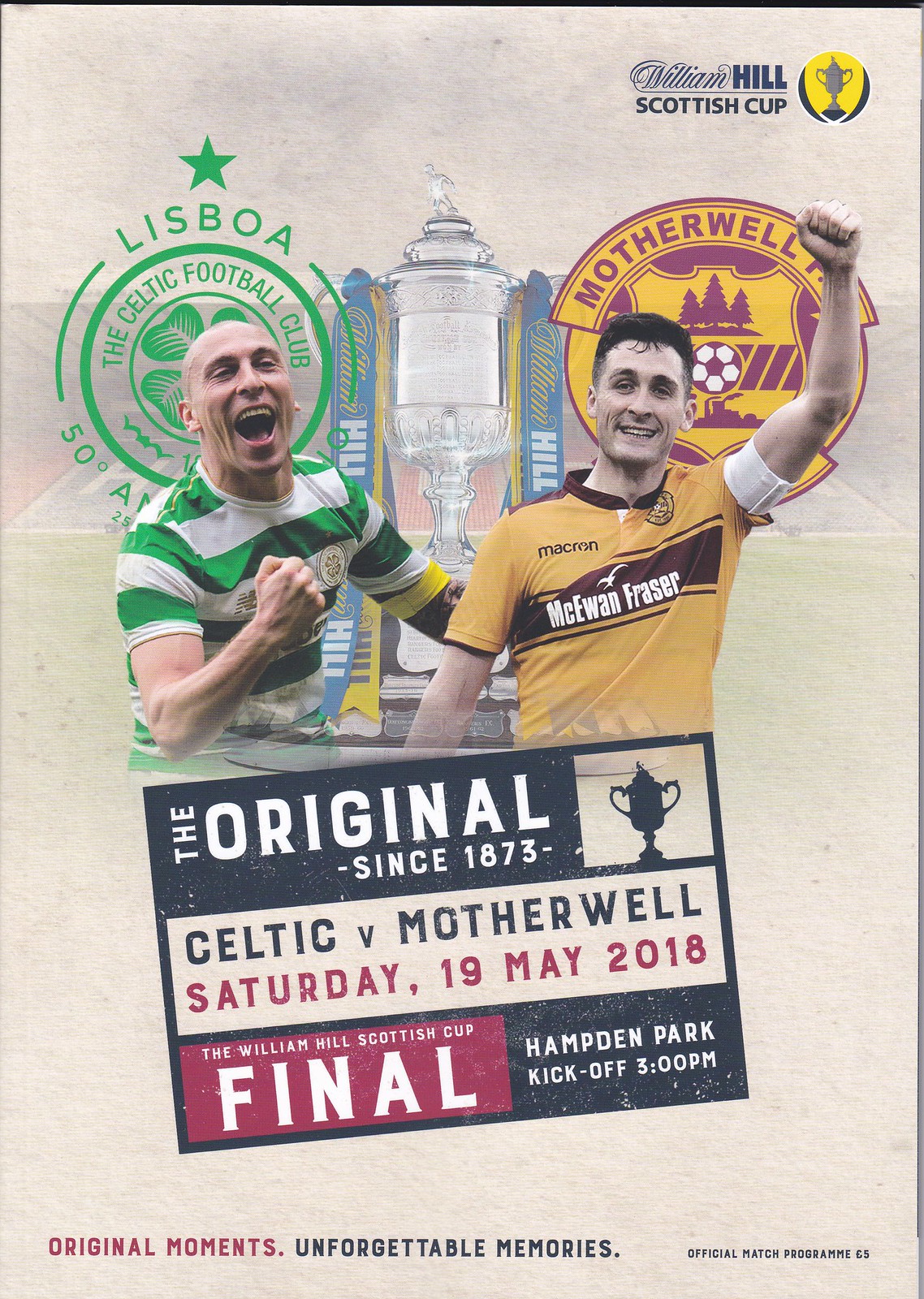The poster, designed to resemble an old piece of paper, announces a match between the Celtic and Motherwell football clubs. At the top, the image features two excited men in their 40s. The man on the left, wearing a green and white striped shirt with the Celtic F.C. logo 'Lisboa' behind him, has his mouth open and his right forearm raised in a celebratory fist. The man on the right sports a yellow and brown shirt with 'McEwan Fraser.' Above him is Motherwell's logo, which includes a soccer ball. Centered between them is a large silver cup with two blue ribbons. Below the cup is a dark blue rectangle with white text: "The Original Since 1873, Celtic vs. Motherwell, Saturday 19 May 2018, the William Hill Scottish Cup Final, Hampden Park, kick-off 3pm." The background of the poster features a stylized photograph of a soccer stadium with a gray filter.